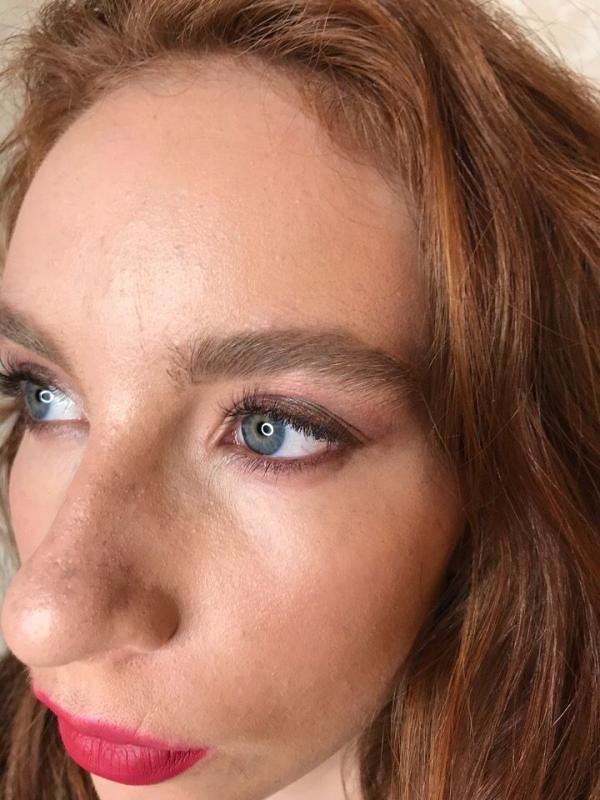This intimately close-up photograph captures the face of a woman, likely in her early thirties, who appears to be of Caucasian or possibly Hispanic descent. The image is taken from a slightly elevated angle, focusing tightly on her face as it turns toward the left, revealing a clear profile. She has striking red hair that appears slightly wavy and pushed back off her forehead, framing her face but not visible beyond her shoulders. Her blue-green, possibly hazel eyes are accentuated with dark eyeliner and eye shadow, paired with curled dark brown eyelashes. The woman's thick, light brown eyebrows frame her pronounced nose, which stands out as her most defining feature. Her lips are vividly painted with red lipstick, and a few faint freckles can be seen across her nose. Despite the presence of makeup, the high-resolution close-up reveals the natural texture of her skin, including visible pores. Her complexion suggests a naturally fair skin tone, with her neck appearing marginally paler than her face. The overall composition emphasizes her facial details, offering a nuanced portrayal of her expressive features.